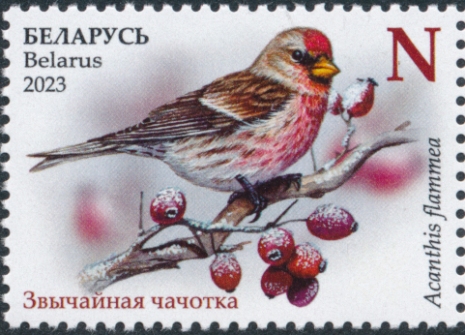The image features a 2023 edition stamp from Belarus. Dominated by a detailed illustration of a bird, the stamp showcases an avian species with a red crest, chest, and head, grayish body, and brown wings. The bird is perched on a branch adorned with red berries, lending a picturesque touch. Along the right side of the stamp, the bird's Latin name, "Acanthus flammea," is inscribed. In addition, the top left corner displays "Belarus" written in Cyrillic script, while the bottom left also includes text in Cyrillic. The bottom right corner contains text in black, and the letter "N" is prominently placed in the top right corner, marking its denomination. The English word "Belarus 2023" is also present, providing an international touch.